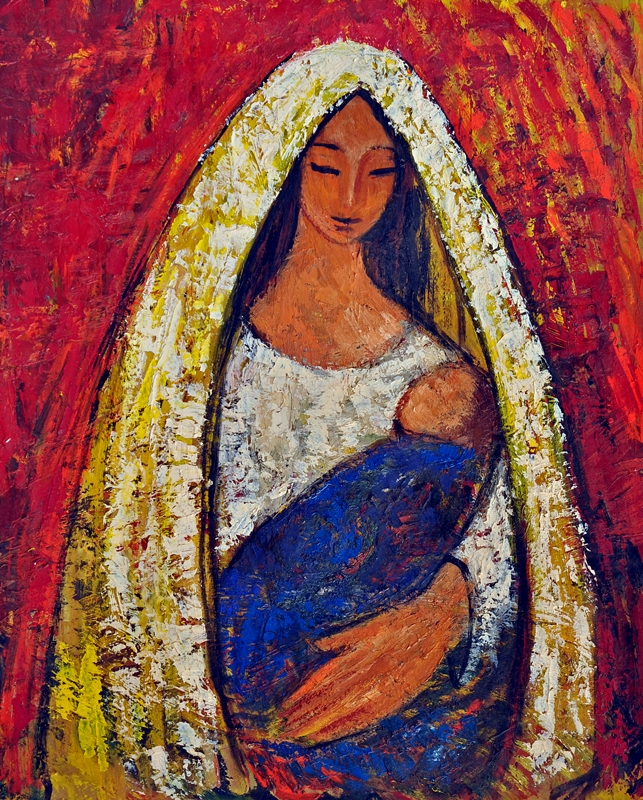This vertical rectangular painting is a non-traditional interpretation of the Virgin Mary holding baby Jesus. The background is a striking, textured red, interwoven with streaks of black, blue, orange, and yellow, producing a vivid and dramatic effect. Central to the composition is a woman with tanned skin, an oval-shaped face, and brownish-blackish-bluish hair that falls elegantly behind her. She gazes down at the child in her arms, her eyes appearing as narrow black slits.

The woman is wearing a white scoop neck top, accented with hints of tan. Draped over her head and cascading over her shoulders in a protective, cape-like manner is a striking gold and yellow veil, which forms an oval that comes to a point at the top, effectively cocooning her within its embrace.

The infant, swaddled in a deep blue blanket that extends beyond the frame of the painting, rests in her right arm, which supports him with a noticeably long hand. The baby's face is indistinct, rendered in an orangey tan hue, matching the woman’s skin tone.

Overall, the image combines traditional religious iconography with vibrant, modern artistic techniques, resulting in a stunning, evocative portrayal.